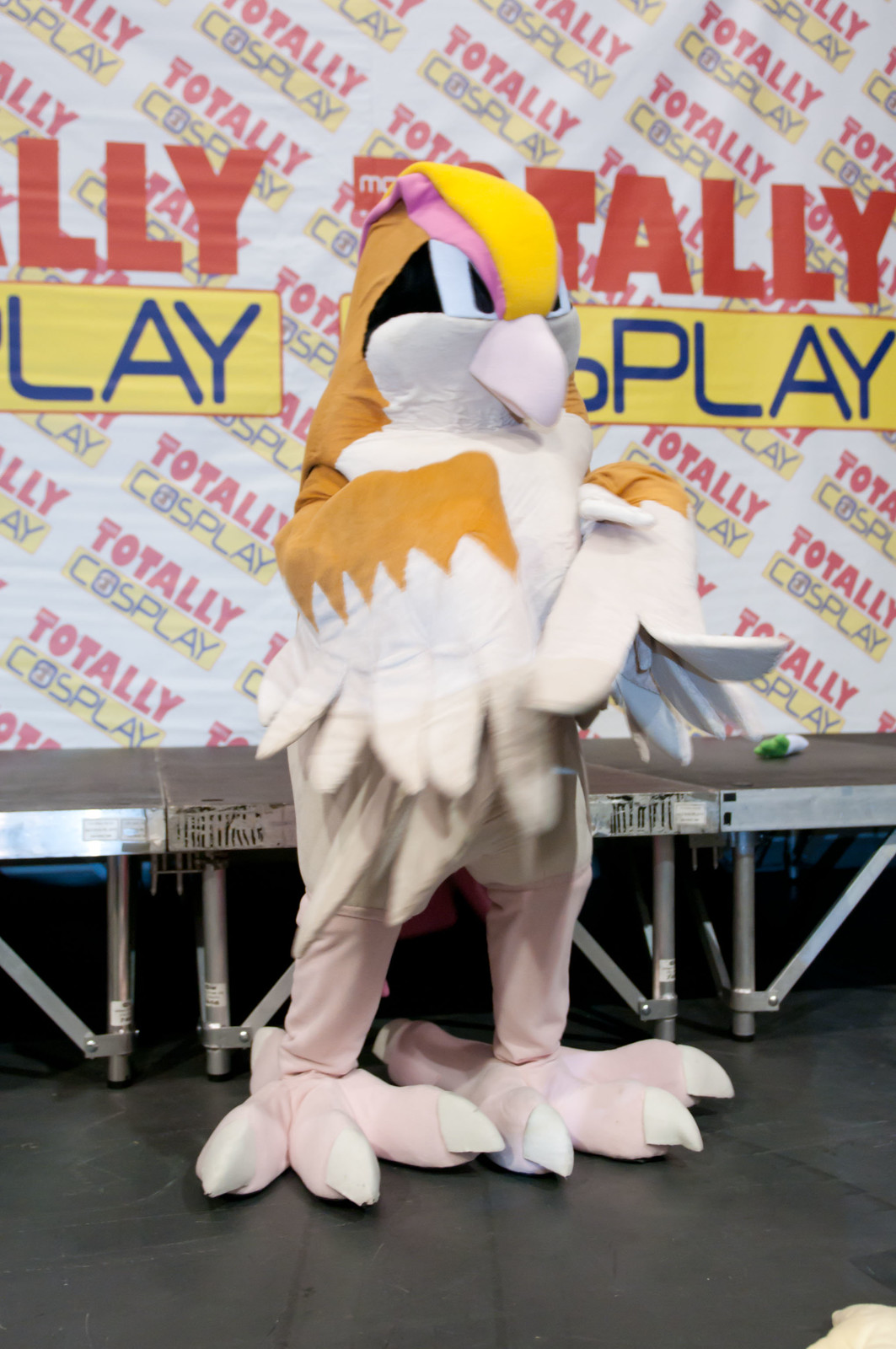The image features a person dressed in a full-body bird costume, likely of the Pokémon Pidgeotto or Pidgeot. The costume, predominantly off-white with beige undertones, includes distinct features like wings and talons, with a yellow and pink crest on the head, black and white eyes, and orange accents on the wings and head. The feet of the costume appear beige with a slightly pinkish hue, ending in white nails. The individual is standing alone on a small stage with metal legs, in front of a backdrop that repeatedly reads "Totally Cosplay." The words "Totally" are in large red letters, while "Cosplay" features a yellow background with blue writing. This text is prominently displayed behind the performer, enhancing the theme of the event.